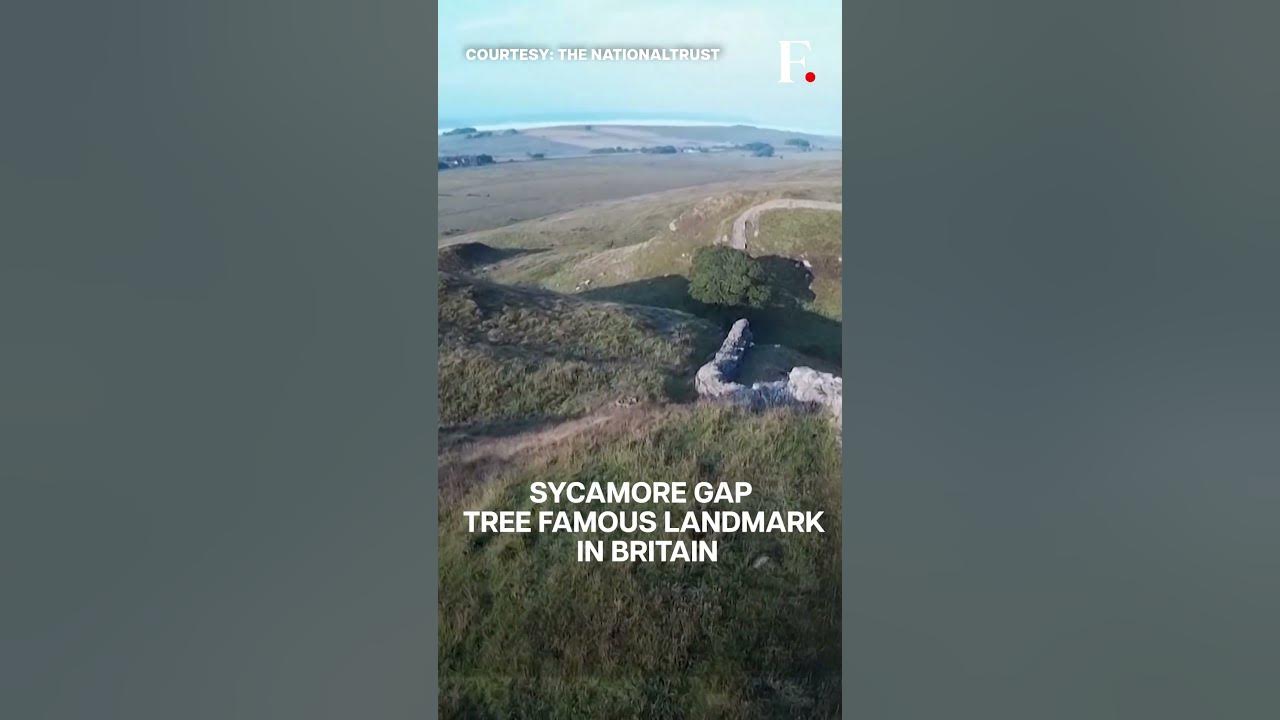The image depicts an outdoor landscape captured from an aerial perspective, showcasing a wide expanse of green grass interspersed with pathways and walkways, dotted with trees and bushes. A prominent feature is the Sycamore Gap Tree, a famous landmark in Britain, which casts a distinct shadow on the ground. The text at the top of the image reads, "Courtesy the National Trust," and in the top right corner, there is a white letter 'F' followed by a red dot. The sky, a light blue with scattered clouds, enhances the calmness of the sunny day. In bold, white capital letters at the bottom, the text "Sycamore Gap Tree Famous Landmark in Britain" is center-justified in a sans-serif font, standing out against the natural scenery. A large rock wall or formation is visible on the right side, partially obscured by the large tree’s shadow. Shadows from the bushes towards the middle of the image further accentuate the landscape's depth and texture.